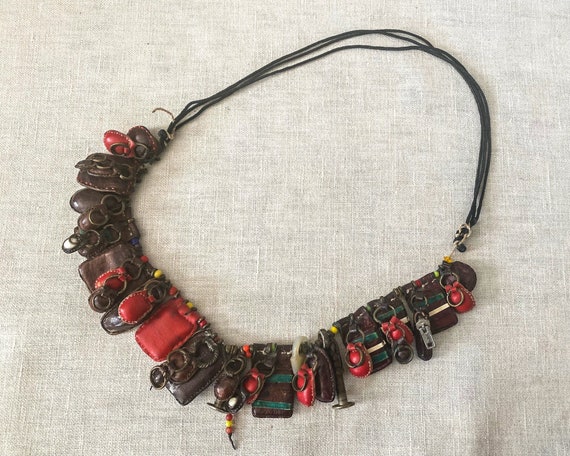The image features a unique and handcrafted necklace, strikingly non-traditional in design. The upper part of the necklace consists of three thin, black cords, messily tied together with visible knots, transitioning into a thicker, beige thread. This beige section is adorned with an eclectic mix of items that give the necklace a distinctly rustic and possibly tribal appearance. There are several leather pieces, predominantly brown, with some red, pillowy pouches, and striped brown tags. Metal elements such as rings and a zipper tag hang from the thread, adding an industrial touch to the otherwise earthy composition. The necklace rests on a beige linen sheet or tablecloth, accentuating its handmade, artisanal charm.